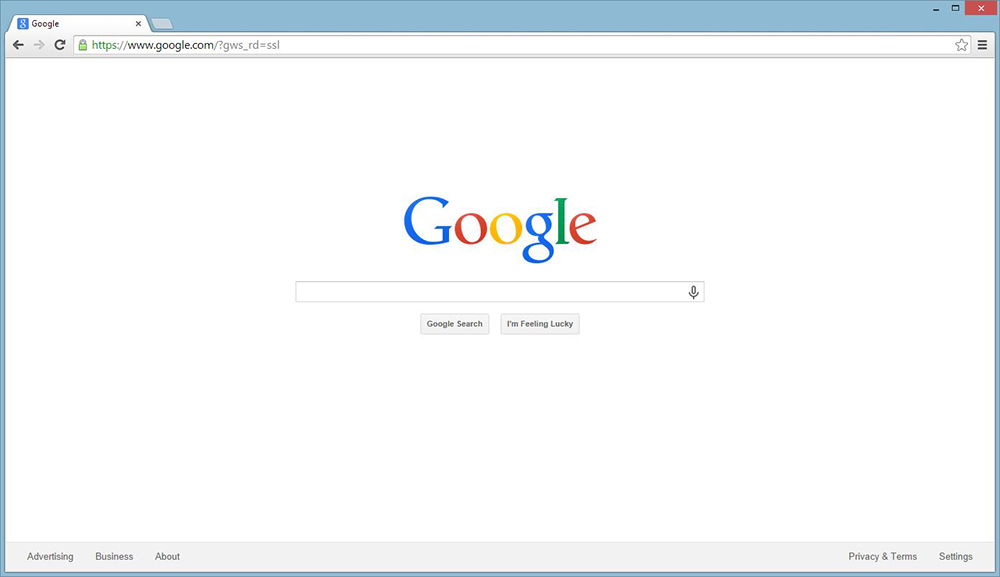This digital image is a screenshot of a computer screen displaying the Google homepage. On the upper left corner of the browser tab, there is a favicon featuring Google's iconic lowercase "g" in blue and white. Adjacent to this, the active tab is labeled "Google." The browser navigation toolbar includes a left arrow for backward navigation, a right arrow that is grayed out (indicating it is inactive), and a refresh button for reloading the page. 

The address bar contains the URL "https://www.google.com," confirming that the homepage of Google is being viewed. To the far right of the address bar, there is an "X" button for closing the tab.

Centrally featured on the screen is Google's multicolored logo: the initial "G" is blue, the first "o" is red, the second "o" is yellow, the lowercase "g" is blue, the "l" is green, and the "e" is red. Below the logo, there are two rectangular buttons: the left one reads "Google Search" and the right one says "I'm Feeling Lucky." Additionally, a microphone icon is present, likely indicating the option for voice search. The design and layout are synonymous with Google's clean and user-friendly homepage interface.